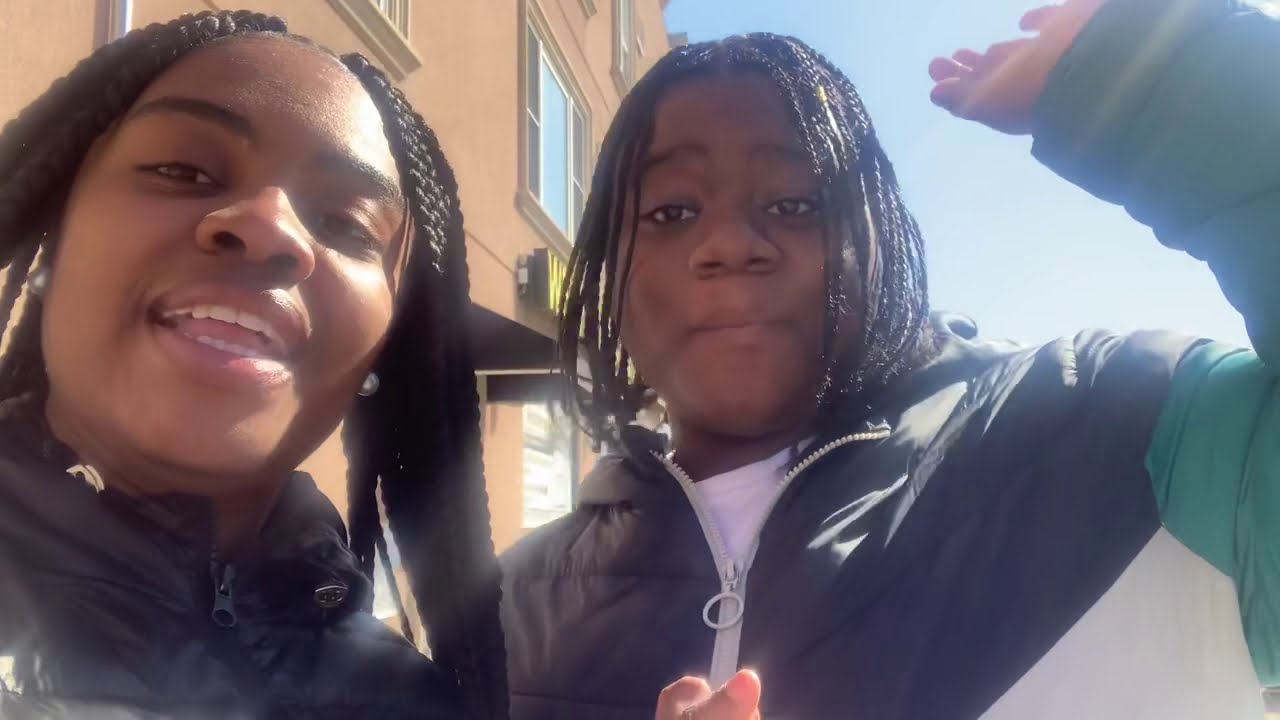This image captures a dynamic moment of two young African American women with braided hair, standing outdoors. Both women are wearing winter jackets, indicating a chilly day. The woman on the left has her mouth slightly open as she seems to be speaking, possibly taking a selfie, showcasing her cheerful demeanor with dark brown eyes and thick cornrows braided down from her head. She is adorned with silver earrings and dons a black puffer jacket. 

To her right, the woman has her left hand raised and is mid-motion, her lips closed as if she is about to say something. Her hair also features black braids that fall to her chin. She is dressed in a multicolored puffer jacket with black across the chest and shoulders, white below, and dark green sleeves, with a t-shirt underneath. 

In the background, there is a clear blue sky and a tall, orange building with at least three floors, providing a contrasting backdrop to their vibrant presence. The overall scene indicates they are standing along the side of a road, capturing a spontaneous and lively moment.